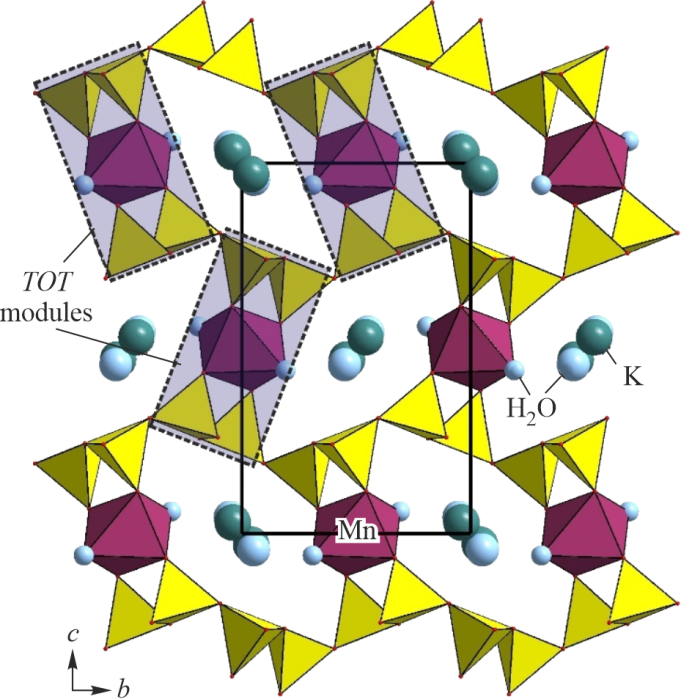The image depicts a complex scientific model known as TOT modules, potentially representing molecules or molecular structures. Central to the image are various three-dimensional geometric shapes, including maroon hexagonal pyramids and yellow triangular pyramids. Interspersed among these shapes are spheres of different colors—dark green, light blue, dark blue, and a light bluish-green. The text within the image labels several elements such as "H2O" for water, "K" for potassium, and "Mn" for manganese. The overall color palette comprises yellows, purples, whites, blacks, and grays with additional accents of light blue and bluish-green. In the bottom left corner, two arrows point upwards and sideways, labeled "C" and "B," respectively, adding to the detailed schematic nature of the depiction.